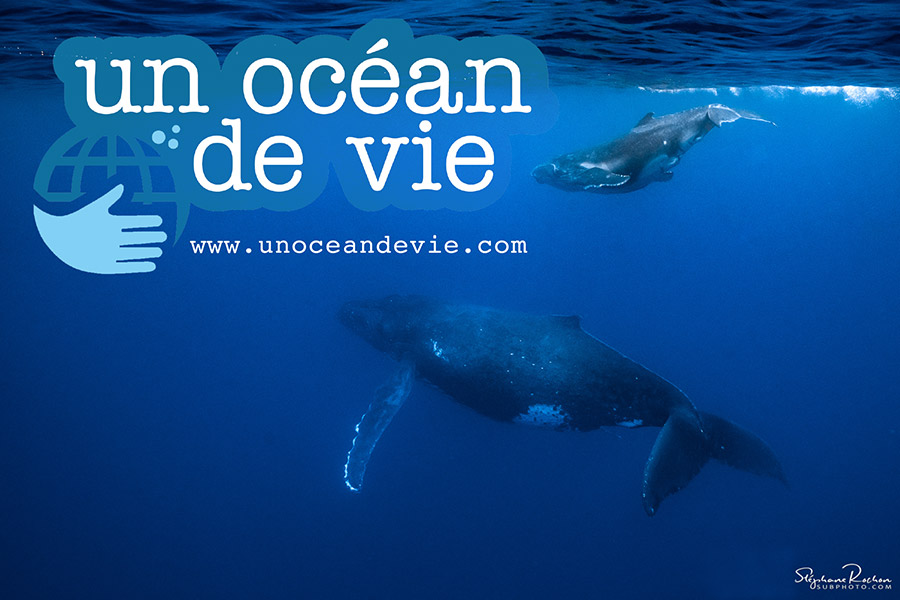The image captures a serene underwater scene featuring two majestic whales swimming in a deep, dark blue ocean. Positioned towards the right of the frame, the whales exhibit a dark blue-grayish hue with distinctive white spots and fringed white edges on their flippers. The surface of the water is just visible at the top, marked by wavy, choppy patterns. In the upper left corner, there's a watermark that reads "Un Océan de Vie" in white text, encased in a thick blue bubble-like highlight. Below this text, there is a light blue globe icon held by a white hand, signifying a logo. The URL "www.unoceandevie.com" is displayed beneath the name. Additionally, a cursive inscription "subphoto.com" in white text is situated in the bottom right corner. The overall impression suggests that this image might be an advertisement or promotional poster for the website mentioned.